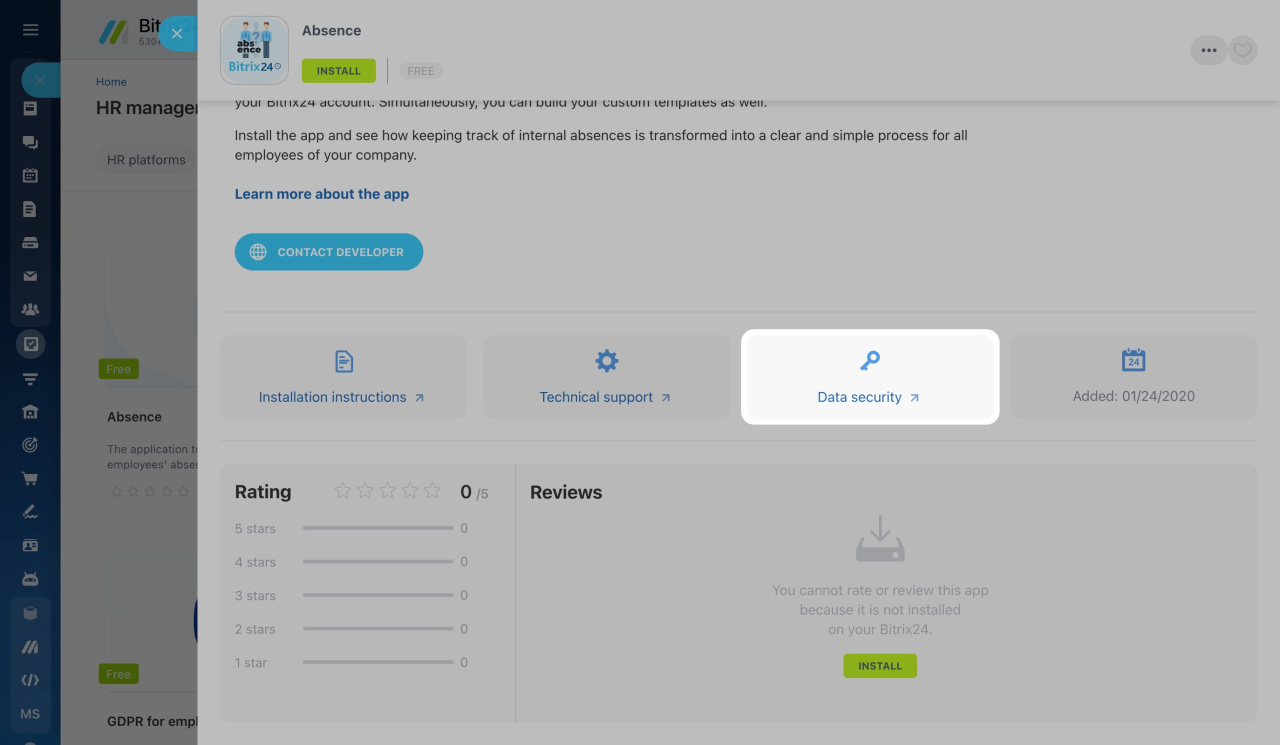This image showcases a Bitrix24 website interface. The main page is partially obscured by a pop-up tab labeled "Absence." The prominent Bitrix24 logo is visible in the top left corner. Beneath the "Absence" title, there's an "Install" button, followed by text explaining the app's functionality: "Install the app to see how keeping track of internal absences is transformed into a clear and simple process for all employees in your company." Below this description, there are links to "Learn More About the App" and "Contact Developer."

Further down, the interface features four horizontal boxes labeled: "Install Instructions," "Technical Support," "Data Security," and an "Added On" date. The "Data Security" section is currently highlighted. In the bottom left corner under "Install Instructions," there's a ratings section displaying a five-star rating system, though it shows no current ratings. Next to this is a reviews section indicating that users cannot rate or review the app unless it is installed on their Bitrix24 account. A button to install the app is also visible below this message.